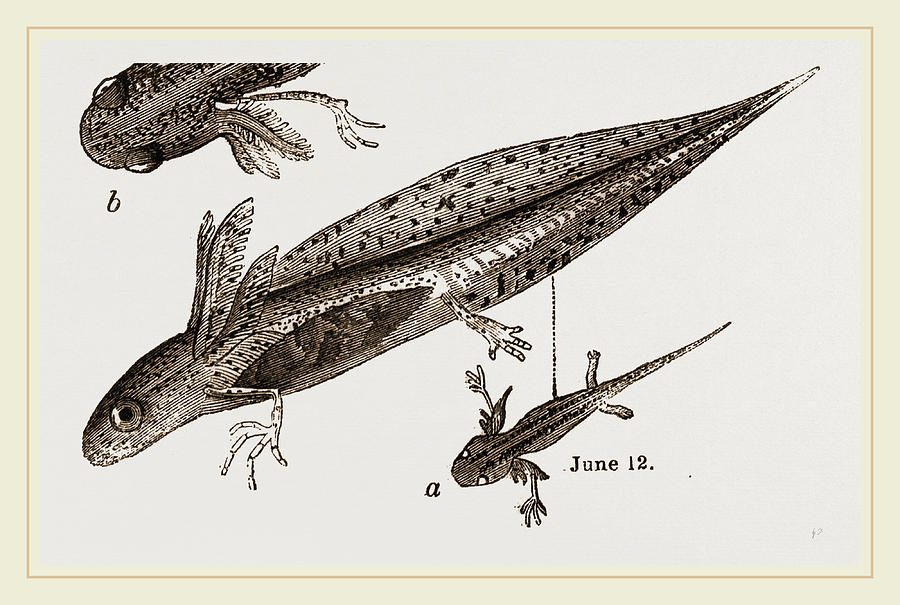The image is a detailed diagram featuring a hybrid animal displayed against a white background bordered by a light brown and gold rim. The focal point of the image extends diagonally from the bottom left corner to the top right, showcasing the animal facing the bottom left. This creature combines features of a fish, lizard, and possibly a tadpole, marked by distinct wings or fins above its two visible left legs. The animal possesses a long, spotted tail and one prominently visible black eye. Above this main depiction, there's a partial top-down view of the same animal, where both eyes and an additional set of three wings are visible, labeled with the letter "B" near the head. Below the main image, there is a smaller view of the creature from above, labeled "A" and also showing both eyes, all four legs, and finer details like black stripes on its body. The date "June 12th" is inscribed underneath this smaller view, suggesting a specific time of observation or annotation.